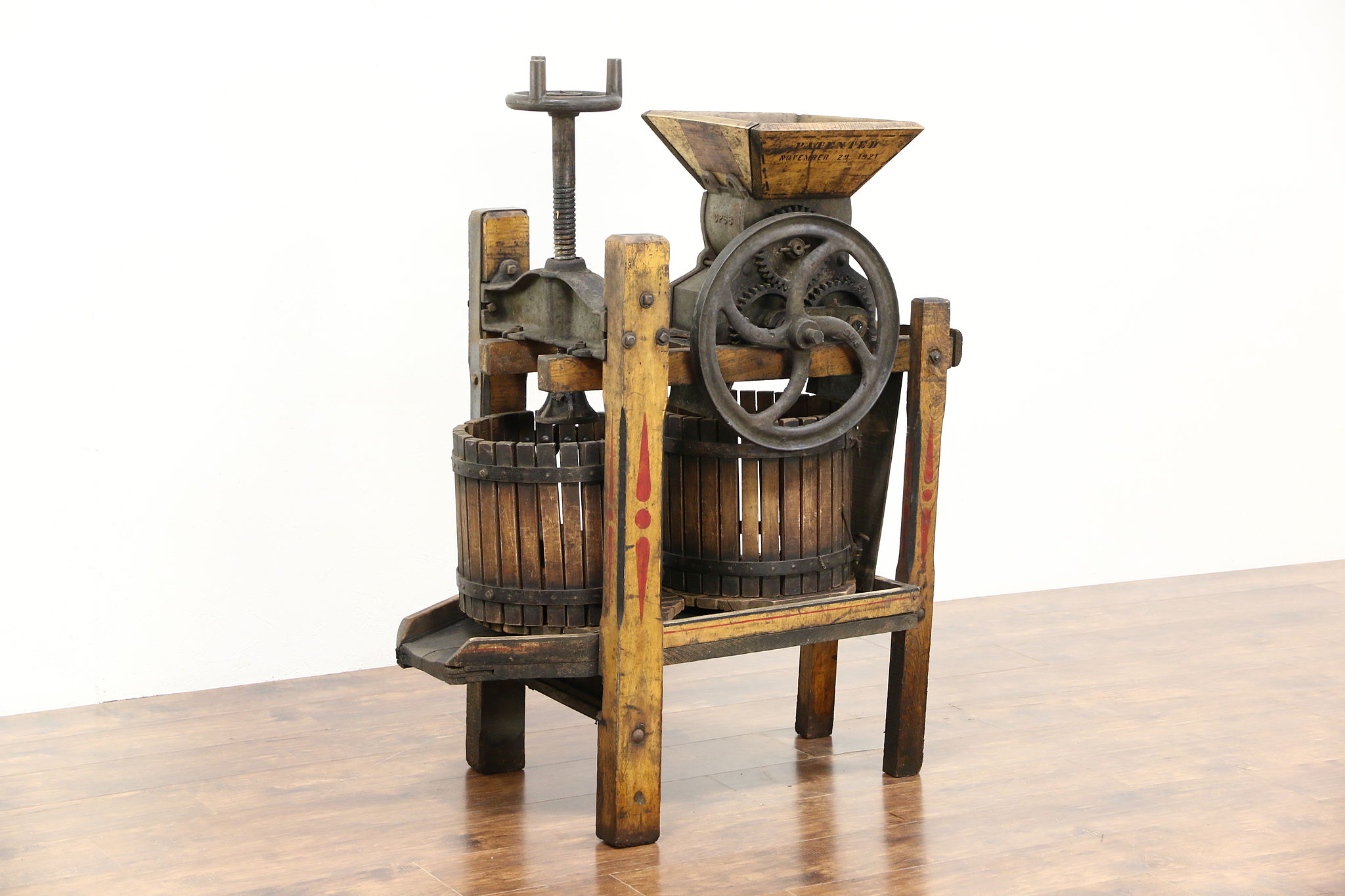This image depicts an old-fashioned apple or grape press, possibly displayed in a museum setting. The press stands on a light brown wooden floor against a plain white background, with a slight hint of light purple in the upper right corner. The contraption is made primarily of wood and features four sturdy wooden legs. It includes a lower shelf that holds two large baskets or buckets. At the top of the apparatus, there is a feeder tube or funnel for inserting produce. A wheel on the side of the press is used to operate the machinery, turning to lower a vice-like metal arm and compress the contents of the baskets below. The press has a distinct square-shaped top and intricate metal gears, contributing to its vintage appeal. It is an intriguing, old-timey artifact, likely reminiscent of those used on farms for making apple cider or grape juice.